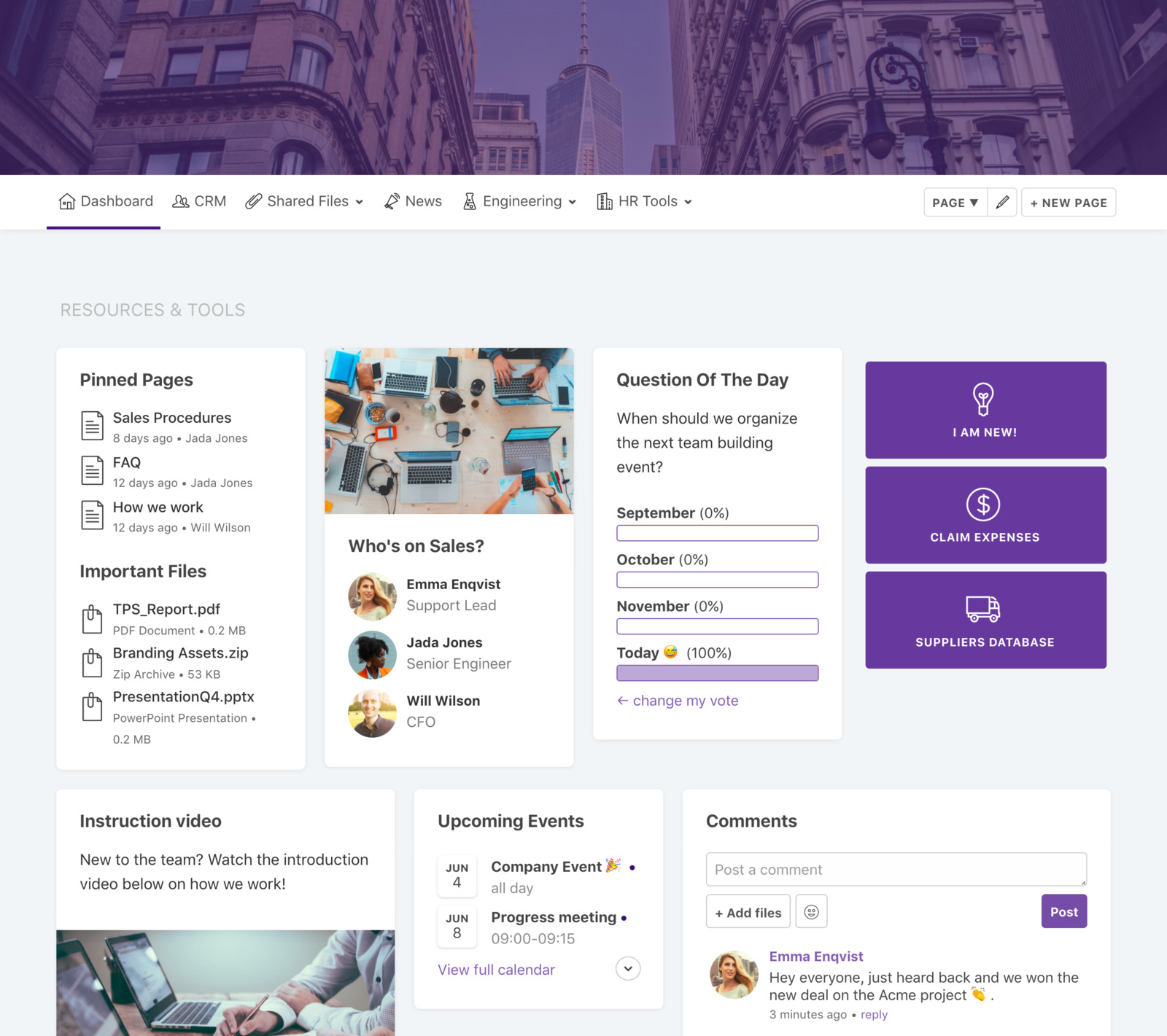The image features a light blue background with a prominent structure at the top—a large box with a darker blue background that showcases a cityscape, towering buildings, and a city corner. Below this, there is a white box containing several elements: the word "Dashboard" underlined in blue, and a list that includes "CRM," "Shared Files," "News," "Engineering," and "HR Tools." Accompanied by these are various buttons—a dropdown menu marked by a down arrow, an edit button symbolized by a pencil, and a "New Page" button.

On the blue background, there's a section labeled "Resources and Tools" which includes a significant white box displaying items like "Pinned Pages," "Sales Procedures," "FAQ," "How We Work," "Important Files," "TPS Report," "Branding Assets," and "Q4 Presentation." 

Centered within the layout is another box with an image at the top depicting people working on computers, accompanied by the text, "Who's on Sales?" It lists the names Emmy Inkvist, Jada Jones, and Will Wilson.

A third white box poses the "Question of the Day," asking, "When should we organize the next team-building event?" with the majority having voted for "today." It includes a purple "Change my vote" button and a left arrow.

Three purple boxes underneath are labeled "I Am New," "Claim Expenses," and "Supplier's Database."

At the bottom of the image, there is an instructional video section with the text, "New to the team? Watch the introduction video below on how we work," accompanied by a picture.

Adjacent to this, a white box lists "Upcoming Events," coupled with a comment box prompting users to "Post a comment." This section also features an "Add Files" button, an emoji icon, and a purple "Post" button. Finally, a comment by Emma is noted at the very bottom.